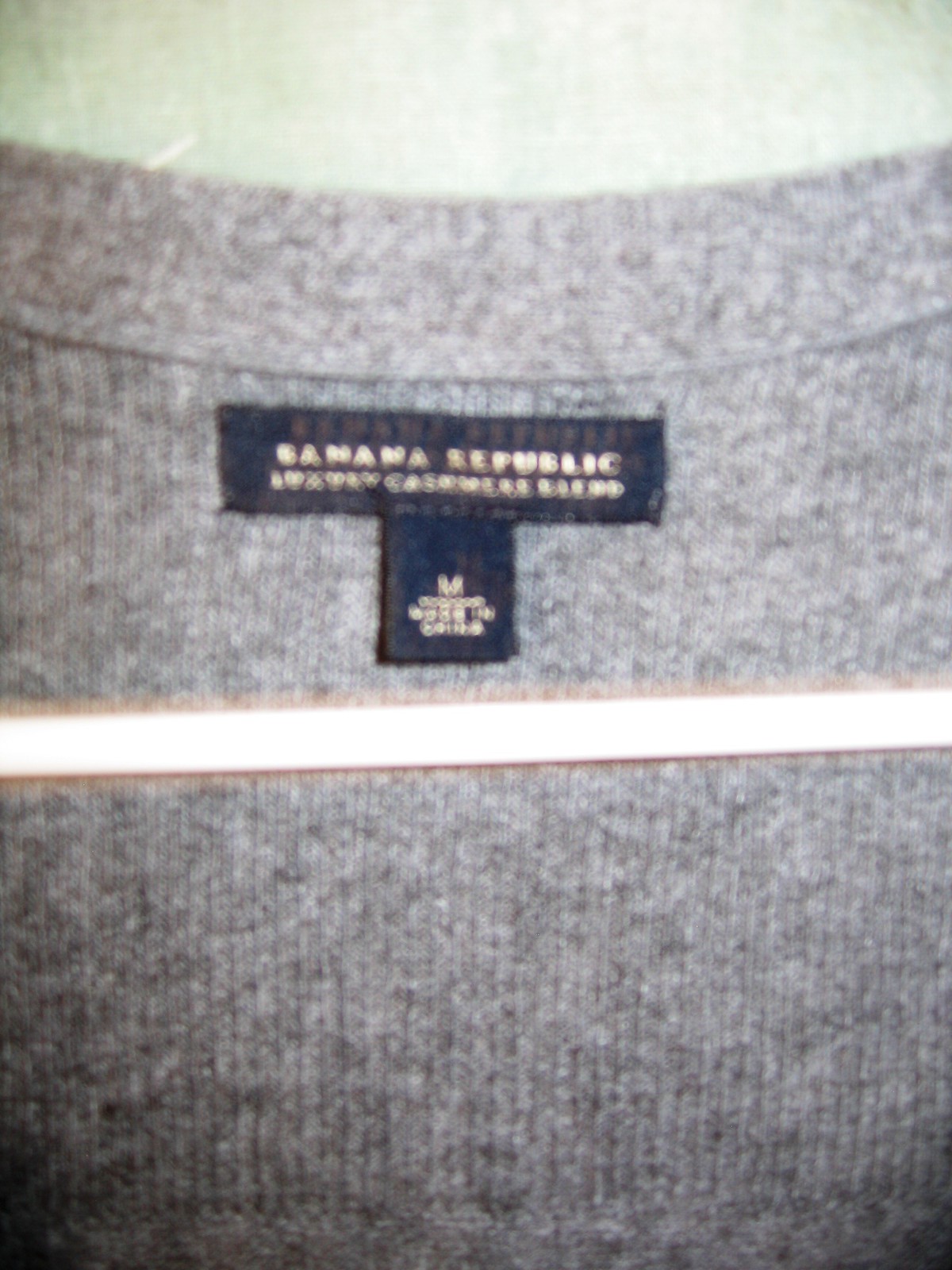The image features a close-up, colour photograph of the back label inside a grey, ribbed sweatshirt, potentially a Henley shirt or sweater. The sweatshirt, speckled with small white flecks, has its tag sewn in just below the collar. The navy blue rectangular label prominently displays the brand name "Banana Republic" in gold lettering at the top, although the text is slightly blurred due to the low-quality, low-resolution capture, possibly from a smartphone held too close to the label. Below this main label is a smaller, nearly square navy tag indicating the size "M" (Medium) in gold letters. A horizontal white stripe, which may be faintly outlined in red, cuts across the shirt, though its exact role—whether part of the design or an element in the foreground—is unclear. The background of the photograph, showing what the shirt is laid upon, appears to be a light green surface.